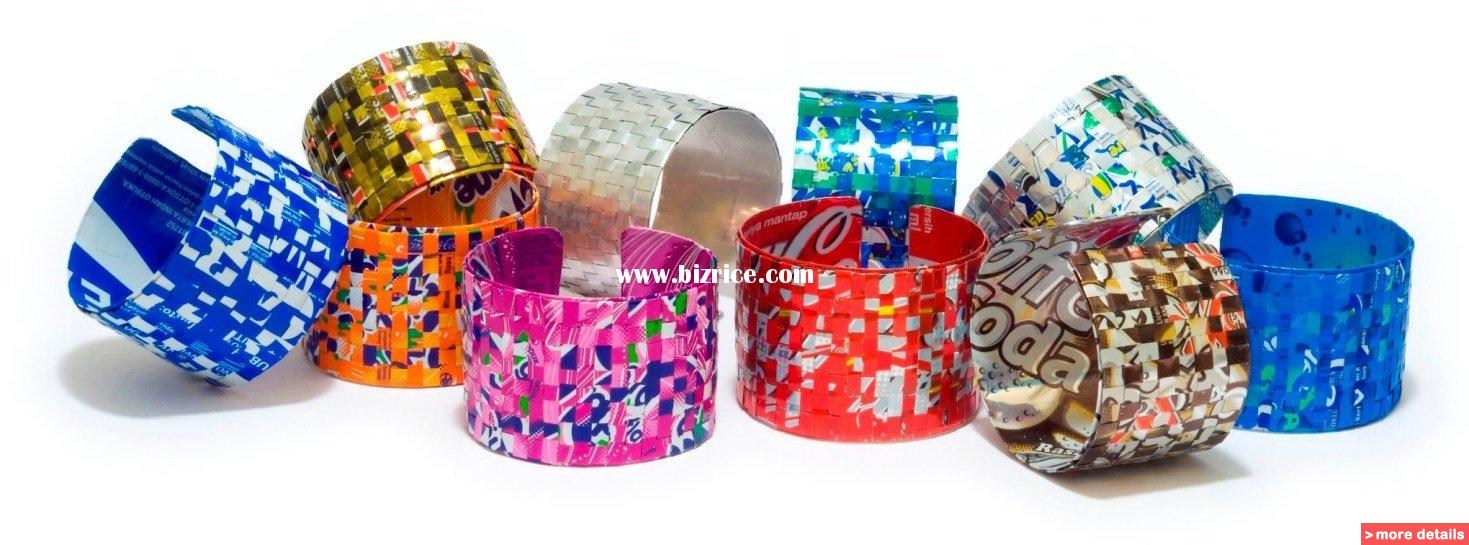This image on a white background showcases about ten wide, bangle-like bracelets made from repurposed soda cans. Each bracelet is open on one side, allowing them to slip onto the wrist. The inner surface of these bracelets reveals fragments of recognizable soda can designs, while the outer surface appears to be covered with a colorful, possibly woven fabric or tape for added comfort and decorative appeal.

Prominent examples include a red bracelet made from a Coca-Cola can, an orange bracelet from a Fanta can, and a bluish-green bracelet from a Sprite can. Other notable mentions are a blue bracelet, an orange and yellow bracelet, and a purplish-pink bracelet. In the center, there is a silver bracelet, and near the back right, another brown bracelet is labeled "coffee soda." The watermark reading "www.bizrice.com" is visible on the image.